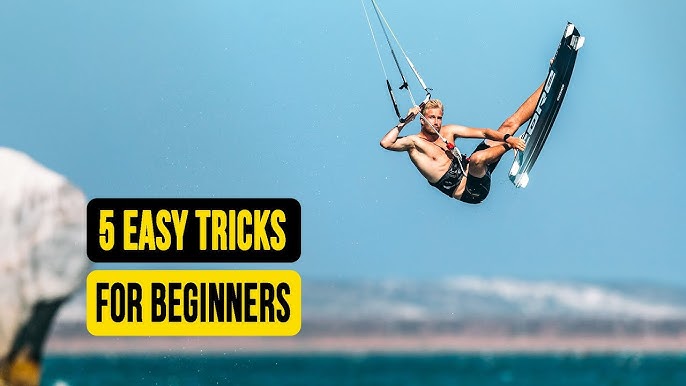The advertisement showcases a shirtless man engaged in parasailing wakeboarding, suspended in mid-air over a vast body of water, likely an ocean. He is equipped with a black strap around his stomach and wearing black shorts. The wakeboard he is using, which features white fins and the word "Core," is securely held in his left hand, while he grips a bar attached to the parasail with his right hand. The vibrant blue sky dominates the top three-quarters of the image, accented by a blurry cliff to the left and distant mountains in the background. In the bottom left-hand corner, two text boxes are prominently displayed: the top box reads "Five Easy Tricks" in yellow on a black background, and the box below it says "For Beginners" in black text on a yellow background.